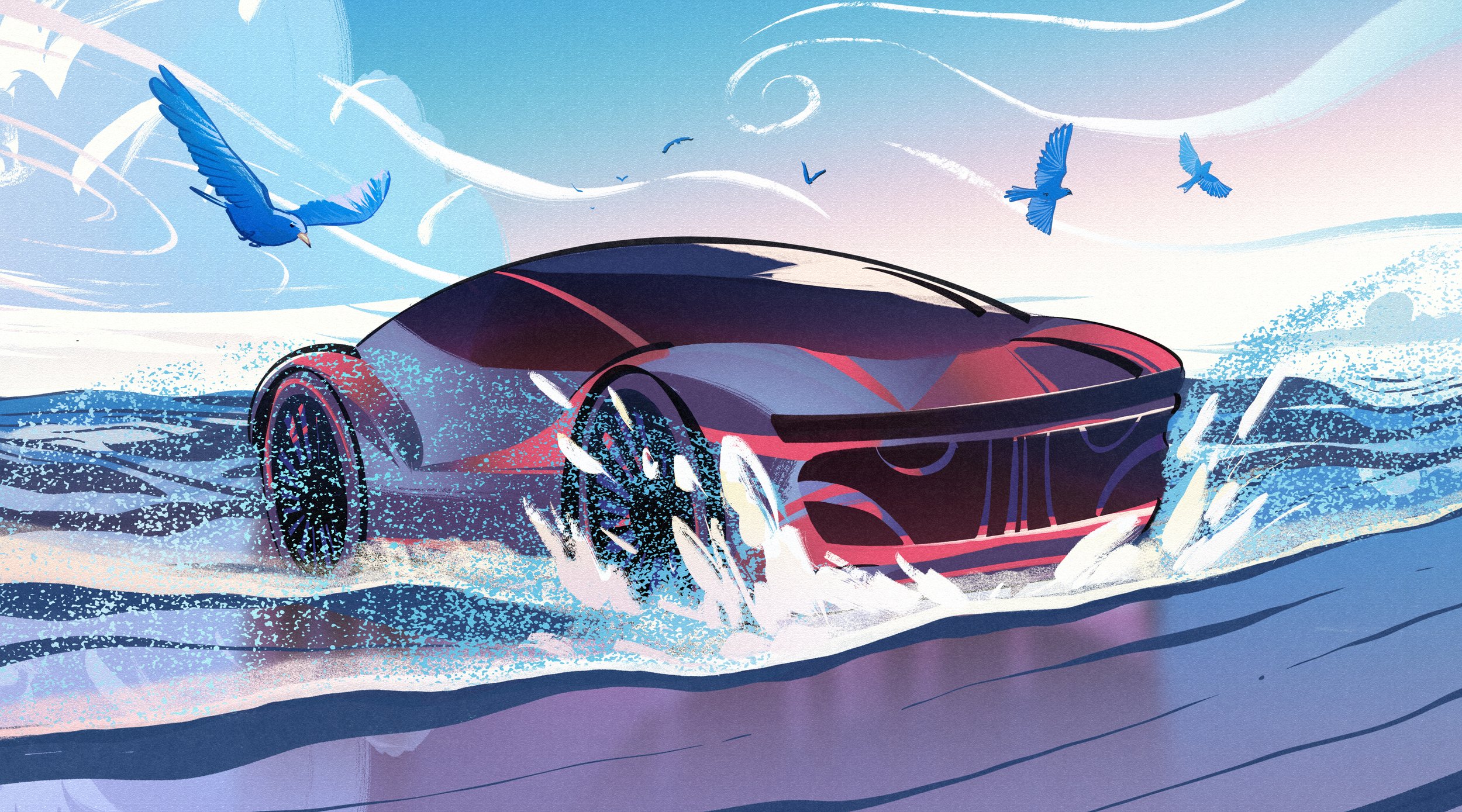This computer-generated image depicts a futuristic sports car driving out of the ocean onto a purplish beach. The car is viewed at a diagonal angle, showcasing its sleek, modern design, with a prominent domed glass top, a giant grill, and four close-set, smooth-lined wheels. The dark purplish-gray vehicle, accented with dark pink, is splashing through shallow blue water, creating dynamic white splashes around its tires. Above, the sky transitions from blue to a light pink hue, adorned with wavy lines representing wind. Blue-hued seagulls, including one detailed seagull in the foreground, fly around the scene, adding a sense of motion. The overall color palette consists of blues, purples, and pinks, giving the image an ethereal, otherworldly atmosphere.